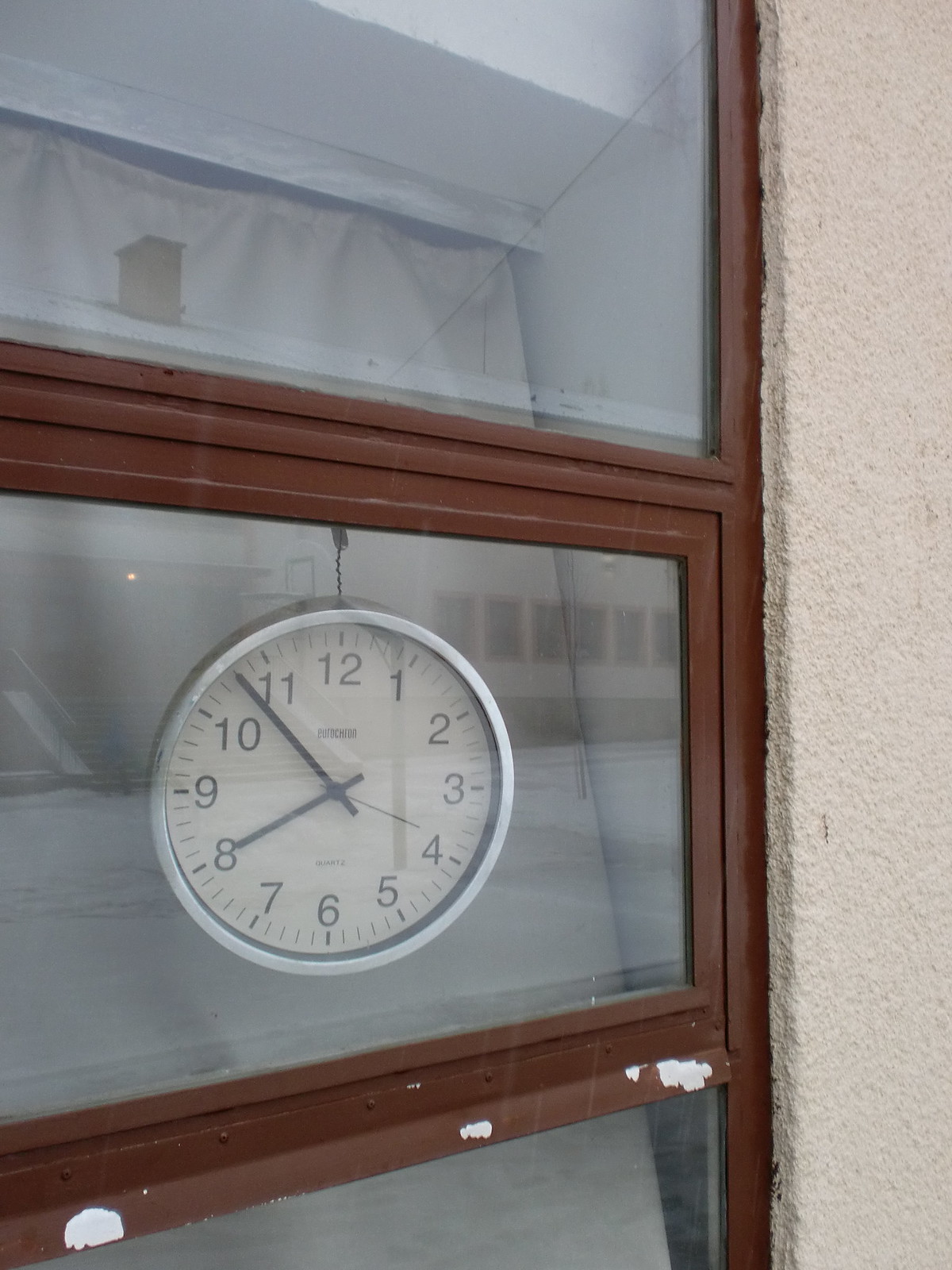This outdoor photograph captures a section of a white stucco building with a prominent brown-framed window that includes three visible glass panes. The window is detailed with chipped paint on the sill, revealing white patches. In the middle pane, a round, silver-framed analog clock hangs from a dark metal wire. The clock features a white face with black hour and minute hands, a red second hand, and black numerals from one to twelve. The time displayed is 7:53 and 19 seconds. Although some text is visible under the twelve, it is indistinct. The reflection in the window captures a glimpse of a building across the way, while a tan curtain hangs behind the glass, adding a subtle background element to the scene.